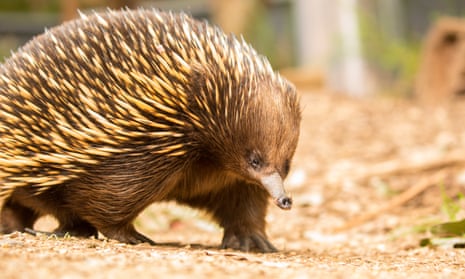In this full-color outdoor photograph, a spiny creature takes center stage, positioned on the left side of the horizontally rectangular image. The animal, possibly a type of hedgehog or an unknown species, features a robust, low-to-the-ground body covered in brown fur. Highlighting its distinctive appearance are thick, yellowish quills on its back. Its small, dark eyes are barely visible and nearly the same size as its tiny nostrils on a notably long, thin snout, giving the creature an almost cute demeanor. The creature's short, dark brown legs support its substantial body as it ambles along a light brown dirt path. The background is mostly out of focus, with blurred shades of light brown earth and potential plant life dominating the right side, and hints of green and gray filling the upper portions of the image, capturing the bright, sunlit forest floor.